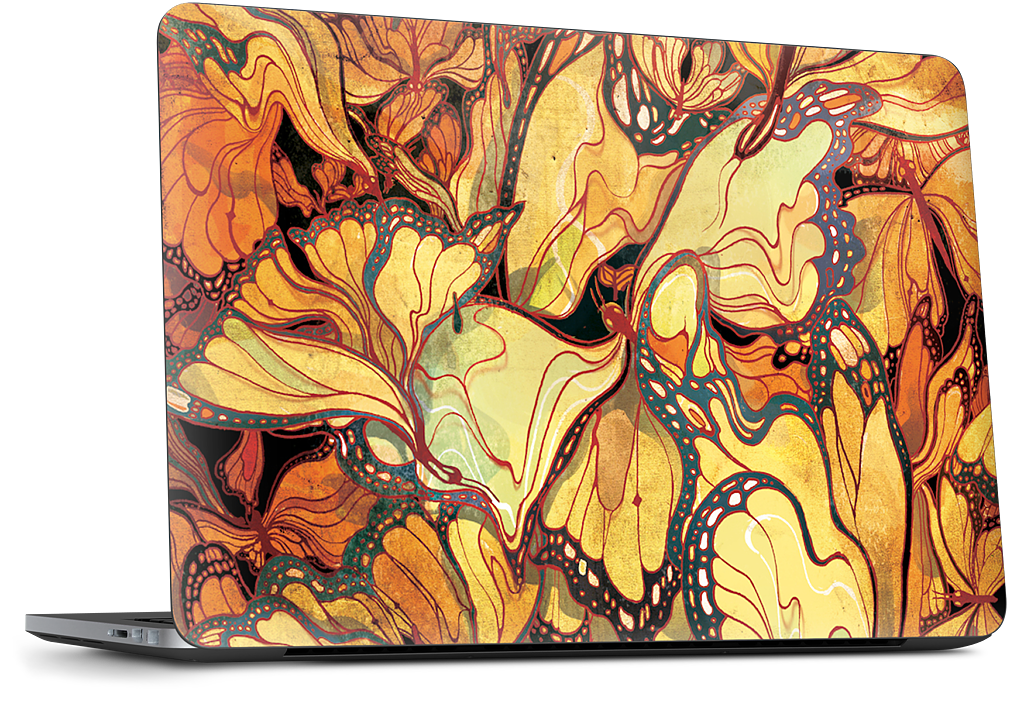This image showcases the back of a metallic silver Apple MacBook, likely a MacBook Air, set against a completely white background. The laptop is partially open at about an 88-degree angle, revealing a small portion of the keyboard and various ports on the lower left side. Dominating the back of the laptop is a vibrant, graphic artwork depicting an intricate collage of Monarch butterflies. The design is layered with multiple Monarch butterflies, their wavy bodies and wings creating an eye-catching and fluid pattern that spans from left to right. Each butterfly showcases varying shades of fall colors, with wings ranging from light yellow to a deep orange, and heads in a burgundy-red hue with tiny yellow eyes. Central to the design is one large, distinctive Monarch butterfly that draws immediate attention. The butterflies have additional detailing with swirly lines and scattered black dots, making the design even more striking and unique.